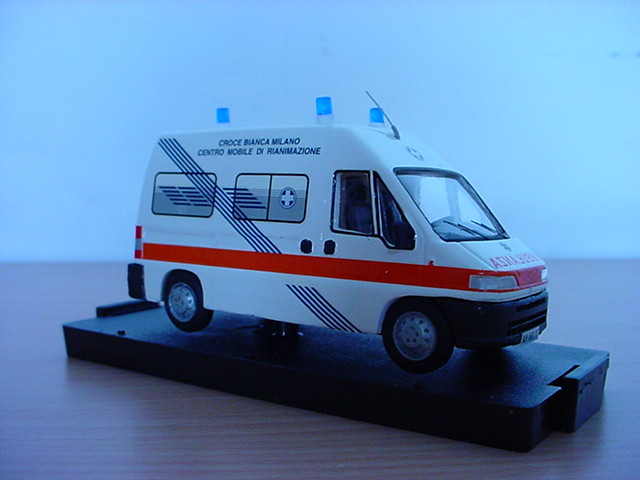This is a detailed color photograph of a white miniature ambulance model, showcased on a black platform atop a wooden table. The image is in landscape orientation with a blue background. The ambulance, which appears distinctly European likely Italian, features an orange stripe around its midsection and a black diagonal line on the side. A red cross emblem is visible on one of the mirrors reflected in the rear window. The vehicle has blue siren lights—two in the front and one in the back—along with a backward-pointing antenna mounted on the roof's front slope. The front and rear of the ambulance are equipped with black bumper guards. Noteworthy details include the Italian text "Grohe Blanca Milano Centro Mobile di Reanimazione" on the side and additional dark blue horizontal striping. The wheels have metallic rims with black tires, adding to its realistic appearance. The photograph does not have any people or text in the background, maintaining focus solely on the detailed model of the ambulance.